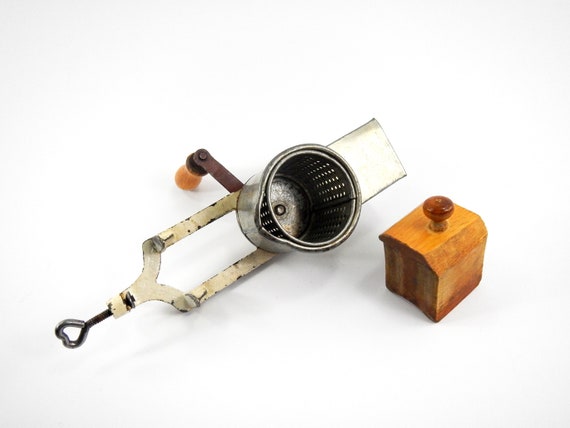The image depicts a vintage-looking cheese grater and a small wooden block on a white background. The cheese grater has a white body featuring a cylindrical grating drum with numerous perforations. A cylindrical chamber is mounted at the top where cheese can be placed, and a crank on the side allows the cheese to be grated through the holes. Attached to the grater is a handle with a brown grip and an orange tip. Beside the cheese grater is a small wooden block, measuring roughly one inch by one inch, with rounded corners and a knob on top, which appears to be constructed from both orange and brown wood. This wooden block seems to function as a pusher for the cheese, aiding the grating process. The scene is set against a plain white backdrop, and the image does not contain any discernible text.